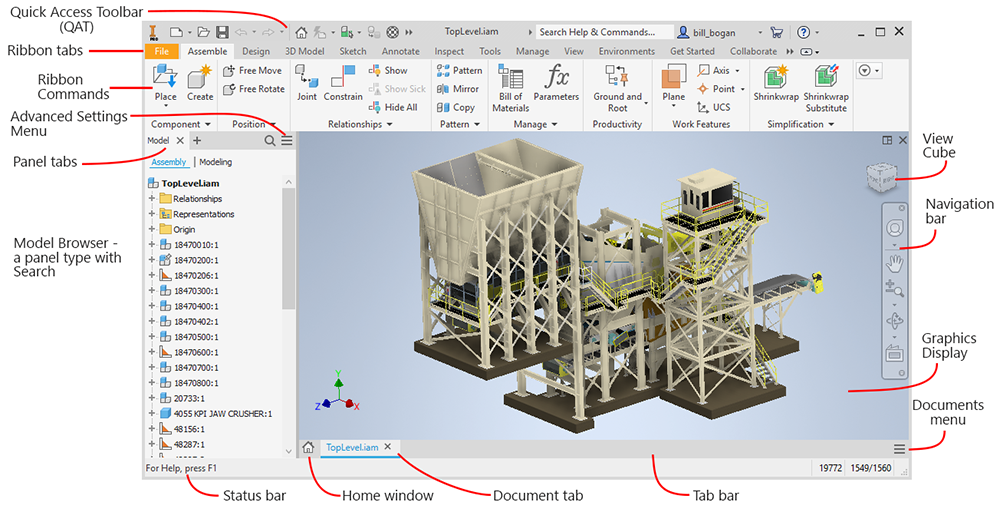This image is a detailed screenshot taken from a computer program designed for 3D modeling, showcasing various labeled interface elements. Dominating the center of the screen is a 3D geometric design of a metal structure under construction. The screenshot features a white background with light grey detailing, emphasizing an organized and clean interface.

At the top of the image, a label with a red line points to the "Quick Access Toolbar (QAT)." Directly below are the "Ribbon Tabs" and "Ribbon Commands," followed by "Advanced Settings Menu," each annotated with precise red-line guides. The left side of the screen displays an indexed panel with labels such as "Panel Tabs," "Model," and "Model Browser," including a "Panel Type with Search."

The bottom part of the screen includes a "Status Bar" with instructions "For help press F1," and a "Home Window" icon resembling a small house. The "Document Tab" is also indicated, leading up to a "Tab Bar" and "Documents Menu."

In the lower right corner, the "Navigation Bar" is annotated, pointing to a blue bar featuring icons like a magnifying glass, a hand, and a "View Cube" for orientation, further detailed with red lines highlighting their locations. The meticulous red-line annotations and black text labels provide an informative guide to all interface elements, making it clear and systematic.